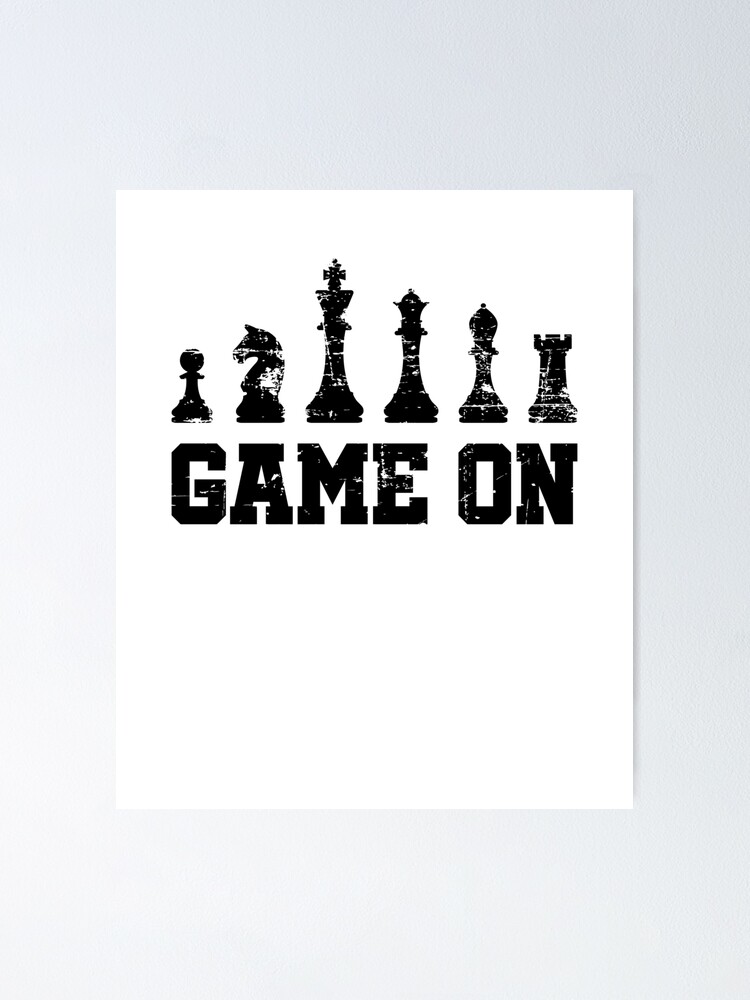The image is a detailed, portrait-mode photograph featuring a central white square card set against a gray background. The card prominently displays the phrase "GAME ON" in a distressed, black print style, suggesting a nostalgic or vintage aesthetic. Above each letter of "GAME ON" are several silhouetted chess pieces arranged in specific order. The pieces include a pawn, a knight facing left, a king, a queen, a bishop, and a rook. The distressed print style reveals white streaks through both the text and the chess piece silhouettes, giving it a sketch-like appearance. This image, with its minimalist yet detailed design, appears to be an invitation or announcement for a chess game, suitable for enthusiasts to possibly display on a wall or use as an invitation to a chess match.